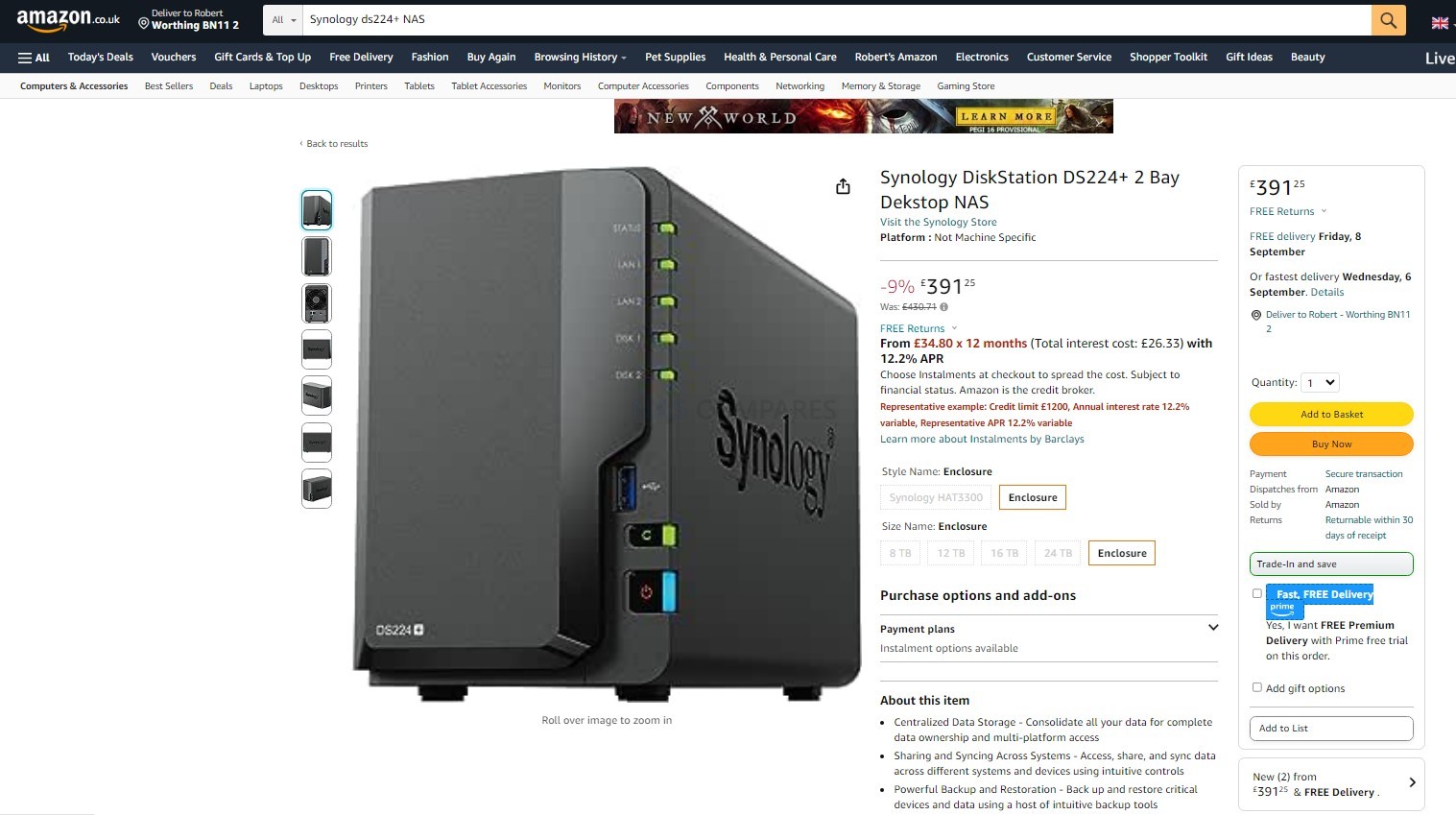This image shows a screenshot of the Amazon UK website (amazon.co.uk), centered on a product search for the Synology DS224+ NAS (Network Attached Storage) device. The familiar Amazon interface is displayed, complete with a search bar at the top center of the page where "Synology DS224+ NAS" has been entered. The search results prominently feature the Synology DS224+, an external data storage system, depicted in a clear, high-resolution product image.

The Synology DS224+ is showcased in its packaging, highlighting its brand name prominently on the box. The device itself, visible in the image, has five green indicator lights on the right-hand side of its front panel. These lights indicate the operational status of the device, varying depending on whether it is powered on or off. Additionally, there is a smaller green light towards the bottom of the front panel, along with a teal-colored power button.

Various functional elements of the Amazon webpage surround the product image, including clickable areas for options like product price, "Add to Basket," and "Buy Now." These elements allow potential buyers to proceed with their purchase easily.